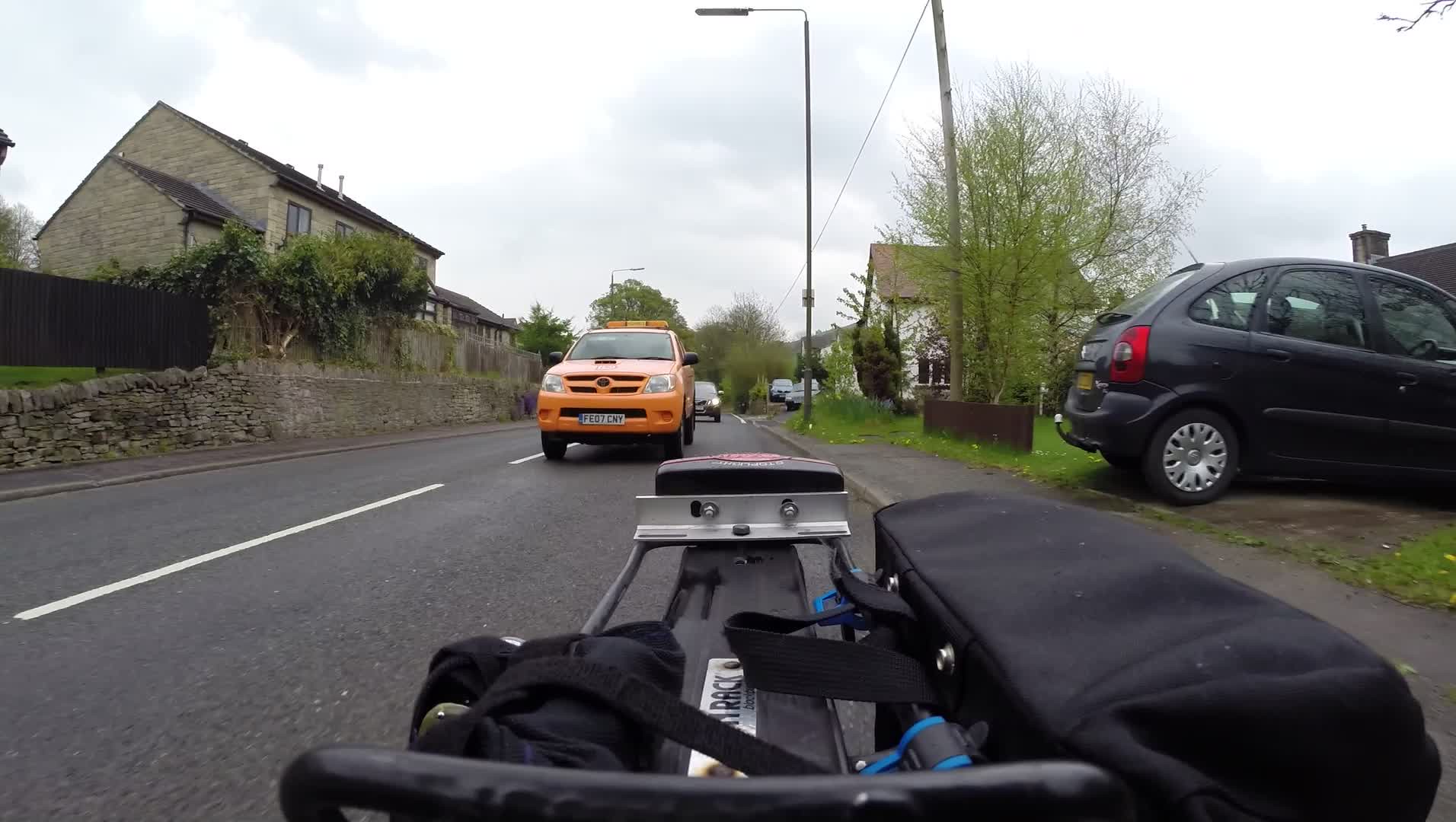In this detailed outdoor photograph, we find ourselves on a tranquil residential street made of smooth asphalt or blacktop. Flanked on either side by charming homes, the street is bordered by clean, well-maintained sidewalks and lush greenery, creating a serene suburban ambiance. Several parked cars line the street and driveways, adding to the everyday feel of the setting. In the foreground, dominating the immediate view, is a distinctive object that appears to be a luggage rack adorned with multiple pockets or attachments, positioned close to the camera. The perspective from which the photo is taken adds an element of intrigue, providing a unique vantage point that piques curiosity. The image is devoid of any text, allowing the visual elements to speak for themselves.